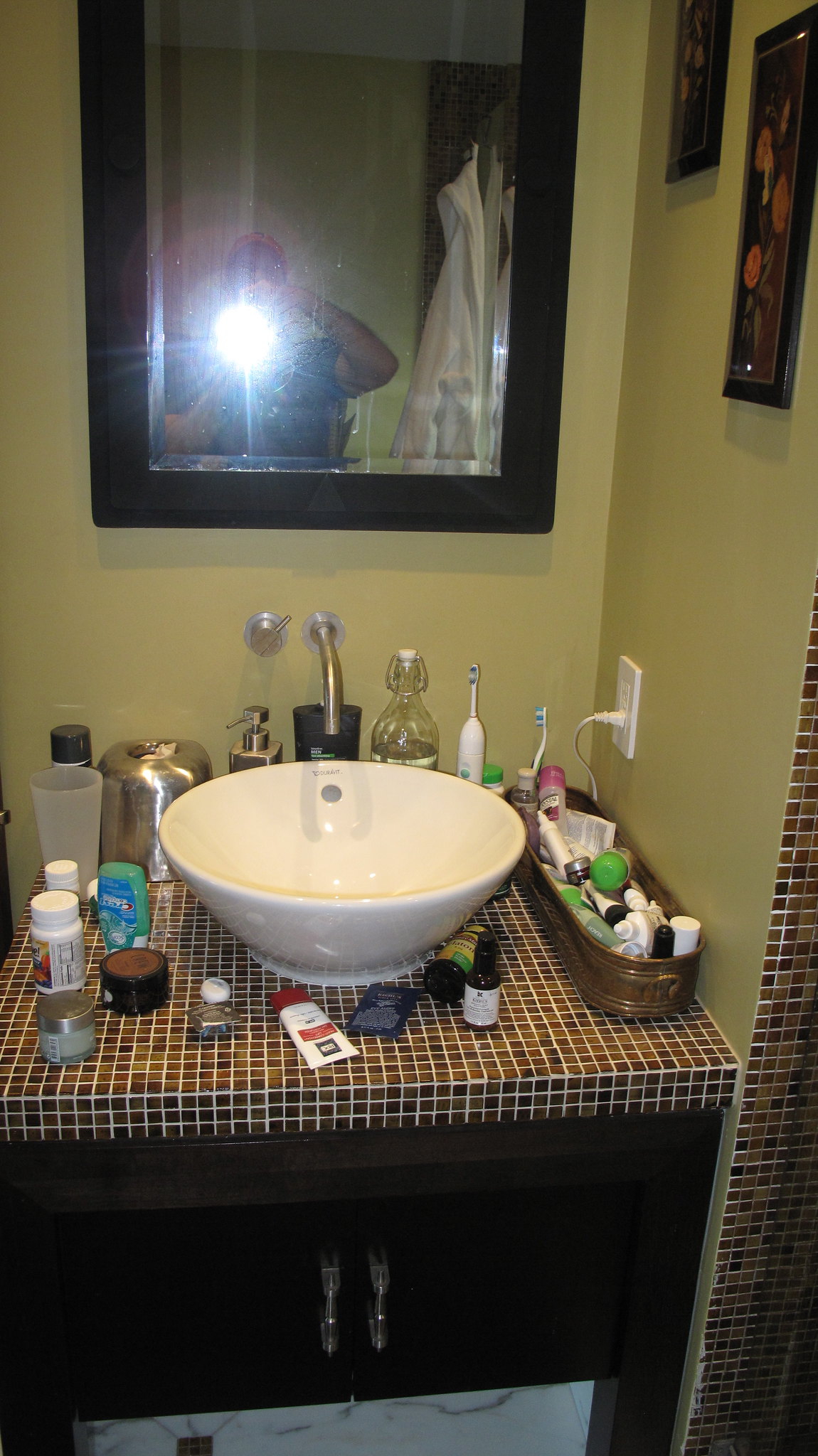The image depicts a meticulously organized bathroom counter with a distinctive brown and white checkered design. At the sink area, there is a prominent bowl-shaped sink that rises several inches above the counter, complemented by a sleek, silver faucet protruding from the wall directly above the white bowl sink. The counter features an array of items, including a white electric toothbrush and several bottles of medicine positioned to the left. A white cup and a bottle of lotion with a red cap also occupy the space, adding to the assortment of personal care products.

To the right sits a long, circular container housing various bottles and products. An electrical outlet is visible with a white cord hanging from it, highlighting the practical aspects of the bathroom setup. The upper portion of the photo reveals a yellowish-green wall, adding a pop of color to the scene. In the center of the wall is a mirror with a black frame, capturing a selfie of an individual whose silhouette is faintly noticeable, marked by a bright flash in the middle of the image. Additionally, two framed pictures are visible on the upper right section of the wall, contributing to the decorative elements of the bathroom.